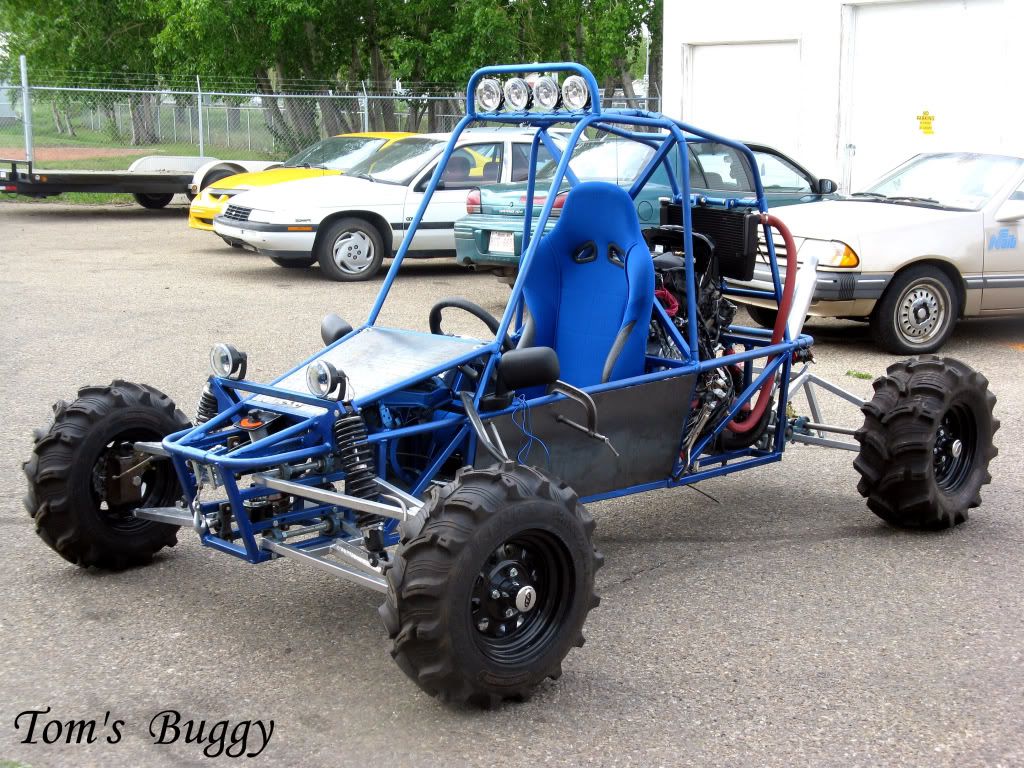This photograph showcases a distinctive blue dune buggy prominently positioned in the center of an outdoor, casual setting. The buggy features a robust blue metal frame, a matching blue seat, and large black tires, with three tires visible from the side angle of the shot. Adorning the top of its cage are four lights. In the lower left corner, black text reads "Tom's Buggy," while a white gradient overlay runs across the lower third of the image, bearing the text, "protect more of your memories for less!" At the top of the image, the watermark "Photo Bucket" is present, slightly obscuring the center. 

In the background, four vintage cars and a trailer are parked: one yellow, one white, one emerald teal, and one tan. The scene is further detailed by a metal fence to the left, a cluster of trees, and some pavement. In the top right corner, part of a white building or garage is visible. The colors in the image span black, white, brown, gray, silver, orange, yellow, bright blue, red, and green, indicating a vibrant and varied palette. The overall setting is unprofessional and casual, taken during daylight, offering an authentic and relaxed atmosphere.